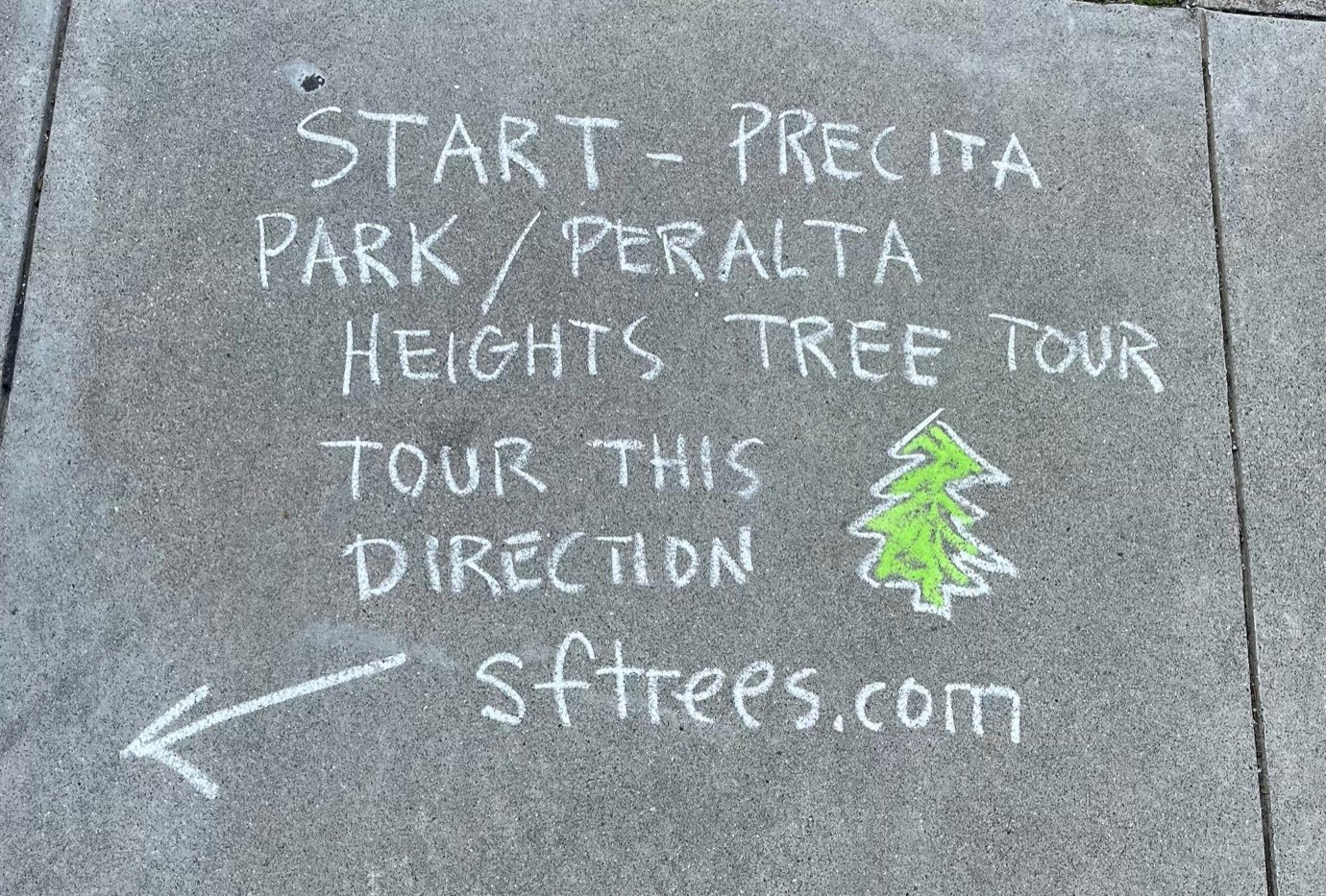This photograph captures a detailed chalk drawing on a gray, speckled pavement with a concrete texture, divided into square blocks by lines. At the top of the image, the handwritten white chalk text begins with the word "Start" followed by a dash, leading to "Precita Park / Peralta Heights Tree Tour" written beneath it. Below these words, the text reads "Tour this direction" with an arrow in white chalk pointing to the left. To the right of the text, there is a small green tree drawn in green chalk with a white outline, resembling a Christmas tree. At the bottom, the website "sftrees.com" is also written in white chalk, providing additional information. The overall scene indicates a clear direction towards a local tree tour in the area.